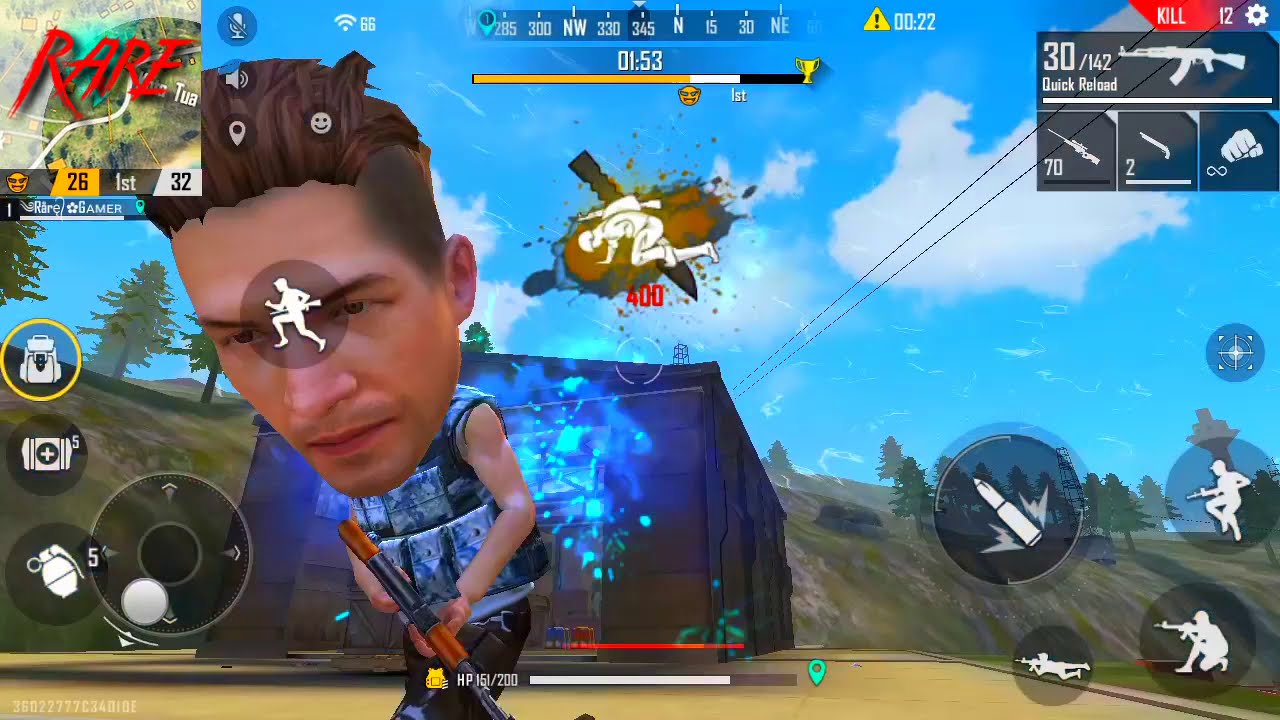The image is a detailed screenshot from an action video game, primarily focusing on a character with a comically oversized head, featuring brown hair that's shaved on the sides and longer on top, along with a bit of facial stubble. The character is wearing a blue or gray bulletproof vest and black pants, holding an automatic weapon. In the background, there's a hill with a shed containing pallets and crates, set against a partially cloud-covered blue sky.

The game's interface is prominently displayed. In the top left corner, the word "RARE" is highlighted in red font. Next to it is an orange smiley face symbol with the number 26, followed by the text "first" and the number 32. Central to the image is a large compass indicating the direction 345, with "north" to its right. Below the compass, a timer shows that there are 1 minute and 53 seconds remaining.

A bar underneath the timer illustrates the player's ranking with an orange section transitioning to yellow and ending in black with a trophy icon, indicating the player's current standing. An exclamation mark in a black circle with a yellow triangle, followed by the number 00.22, is visible at the top right. Another metric shows "kill: 12," indicating the player's number of kills. A settings wheel is located on the right side next to an outline of an AK-47 with ammo details showing 30 bullets out of 142 and a "quick reload" option. Below it, a sniper rifle shows 70 bullets, a shotgun displays 2 bullets, and a fist icon with an infinity symbol is present.

At the bottom left, there's a directional pad for character movement, while five action buttons including a compass, combat poses, and a central shoot button are on the screen. The character depicted appears to be running from a silhouetted figure kneeling beside an explosion with the number "400" in red below them. The bottom of the screenshot features a blue-tinted explosion effect, hinting at combat action, with a building and mountains in the background.